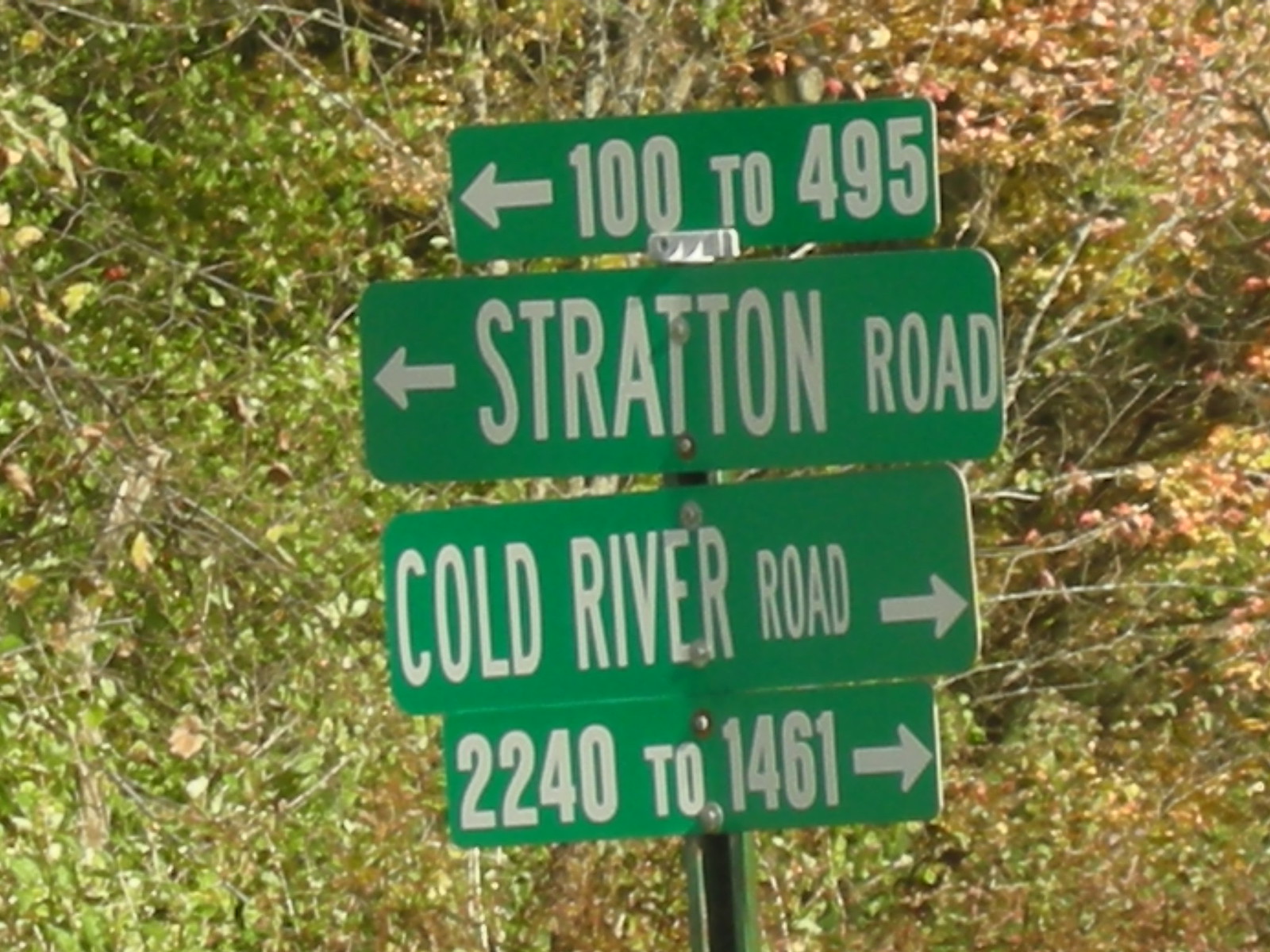This outdoor, color photograph captures a metal street sign post with four distinct green road signs, each featuring white lettering and arrows. The topmost sign directs left and reads "100 to 495." Directly below, another sign also points left and states "Stratton Road." The third sign from the top directs to the right and indicates "Cold River Road." Finally, the bottom sign points right and displays "2240 to 1461." Silver bolts securely fasten each sign to the green metal post. The background reveals a sunny day with a mix of green and brown leaves, suggesting a hint of fall amidst the surrounding trees and bushes.